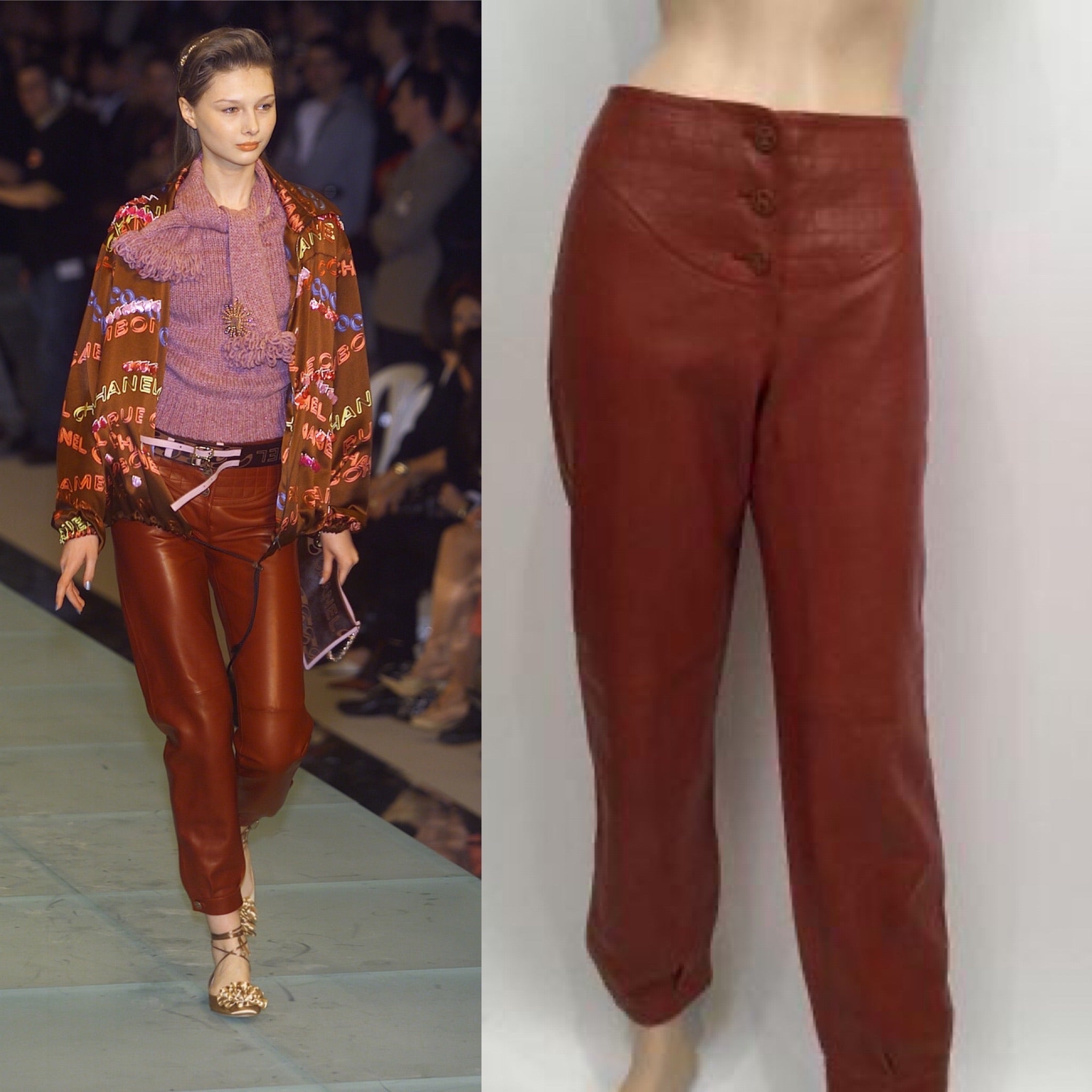The image is a collage consisting of two color photographs showcasing a fashion ensemble. On the left, a fair-skinned model with brown hair is confidently walking down a runway. She is styled in a brown jacket adorned with repeatedly written but indecipherable text in shades of light red and light blue, layered over a pink knit sweater. Her outfit is completed with glossy, red imitation leather pants featuring three small buttons at the waist, paired with gold high heels. She accessorizes with a white belt and a purple and white-bordered handbag in her right hand, while her left hand hangs down by her side. The runway setting is vibrant with spectators blurred in the background watching the fashion show.

On the right, there is a close-up shot of just the red pants, displayed on a mannequin. The mannequin is only visible from the stomach down to the ankles, against a plain white background. The pants, made of a reflective material that mimics leather, are prominently showcased, emphasizing their high-waist design and button details. The quality of the photograph is noticeably inferior to the left, being out of focus and less professional in appearance. This contrast highlights the difference between seeing the garments in a dynamic runway setting versus a static, less glamorous presentation.